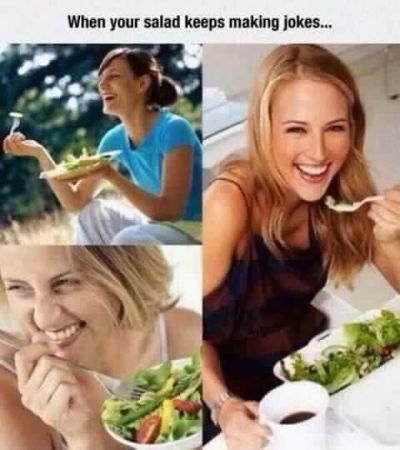The image comprises three color photographs arranged in a square format, accompanied by a gray strip at the top with black text that reads, "When Your Salad Keeps Making Jokes..." On the left side, there are two stacked images: the top photograph depicts a smiling woman with dark brown hair in a ponytail, wearing a blue shirt and white pants, sitting in a grassy field while holding a plate of salad and a salad fork with a piece of lettuce; the background is adorned with trees. Below this, the second image features a blonde woman, seen from the waist up, laughing as she eats a salad from a white bowl, holding her fork with her right hand near her mouth. On the right side, a single vertical image shows another blonde woman with long hair in a black dress, smiling at the viewer while about to take a bite of lettuce off a fork with a bowl of salad in front of her. She also holds a cup of coffee in her right hand, seated against a white background. The overall style is a blend of realism and typography.